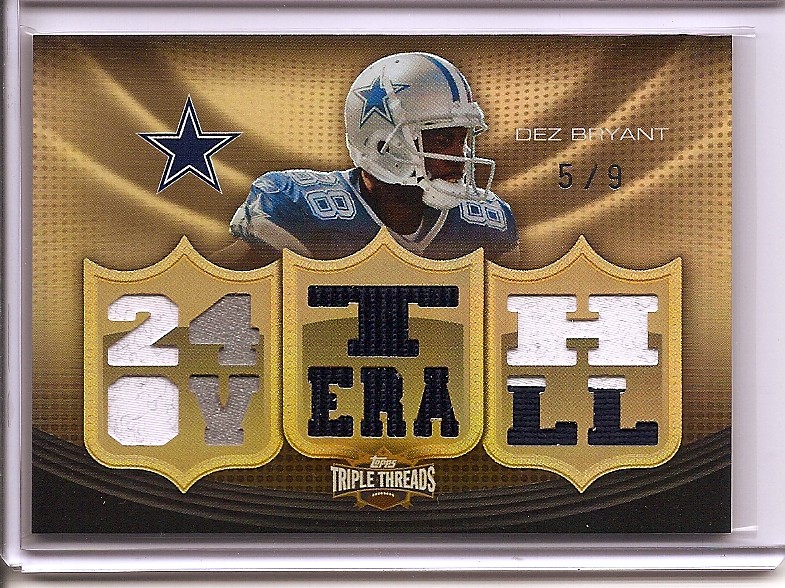The image depicts a limited-edition football collector's card, prominently featuring Dallas Cowboys player Des Bryant. The card has a striking golden background with a small black section at the bottom. At the centre is an image of Des Bryant, showcasing his head and shoulders. He is clad in a blue jersey with the number 88 visible and a white helmet adorned with a blue star on the side. Adjacent to him on the left is another blue star, symbolizing the Dallas Cowboys. To the right, "Des Bryant" is inscribed, along with "5/9," indicating that this is the 5th card out of a total of 9 printed. Below the player's image, there are three golden seals; the left seal reads "24 O Y," the middle one says "T era," and the right one reads "H and then L L." At the very bottom of the card, it proudly states "TOPPS Triple Threads," identifying the brand as TOPPS, renowned for its collector's cards.